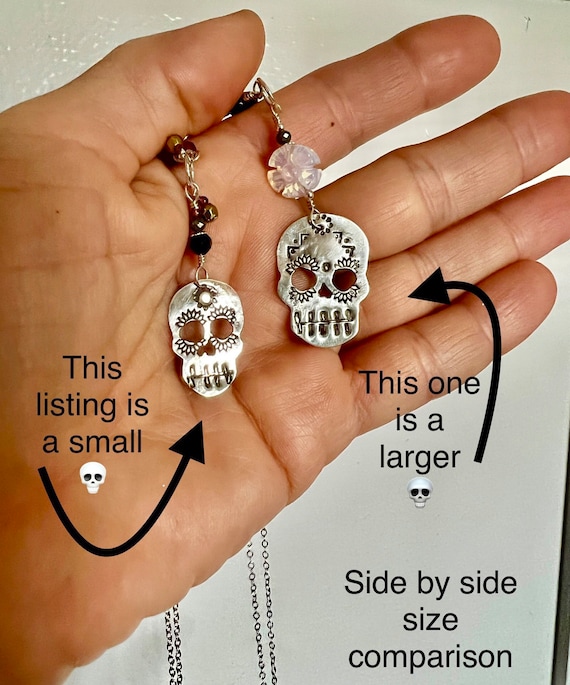The image is a detailed vertical photograph, likely for a listing featuring jewelry items that could be bracelets, earrings, or keychains, all designed with Day of the Dead, or Dia de los Muertos, skull motifs. The focal point of the image is a light brown left hand positioned with the palm facing the camera and fingers pointing slightly towards the top right. The hand is holding two pieces of jewelry—necklaces made of stainless steel with small beads and metal eyelets—each ending in intricately designed metal skull pendants.

Text and arrows in black font are overlaid on the image to provide additional information. On the left side, accompanying the smaller skull pendant, the text reads, "this listing is a small," followed by a skull emoji and an arrow pointing to the small skull. On the right side of the hand, above the larger skull pendant, the text states, "this one is a larger," also followed by a skull emoji and an arrow pointing to the larger skull. At the bottom right corner, there is a label that reads, "side by side, size comparison." The background appears to be a beige wall, possibly with black trim, highlighting the detailed craftsmanship of the skull designs.